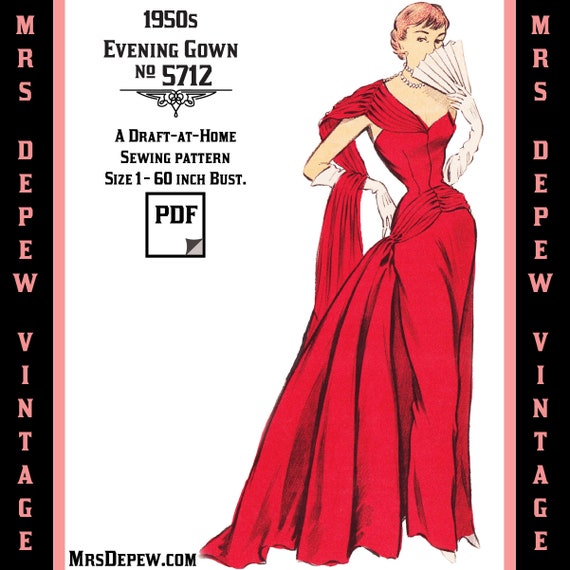The image is a vintage-inspired ad for a downloadable PDF sewing pattern, labeled "1950s Evening Gown, Number 5712," available at MrsDepew.com. The centerpiece of the graphic is a hand-drawn illustration of a woman in an elegant, flowing red evening gown. She has short, pinkish-colored hair and is partially obscured by a white, Spanish-style fan held in front of her face. The gown features a corseted top, a half-cape elegantly draped over one shoulder, and a tight-fitting skirt with a slight bustle at the back. She accessorizes with long, white evening gloves. The ad is set against a white background with black lettering, and the brand "Mrs. Depew Vintage" is prominently displayed in a black background with pink lettering on both sides.